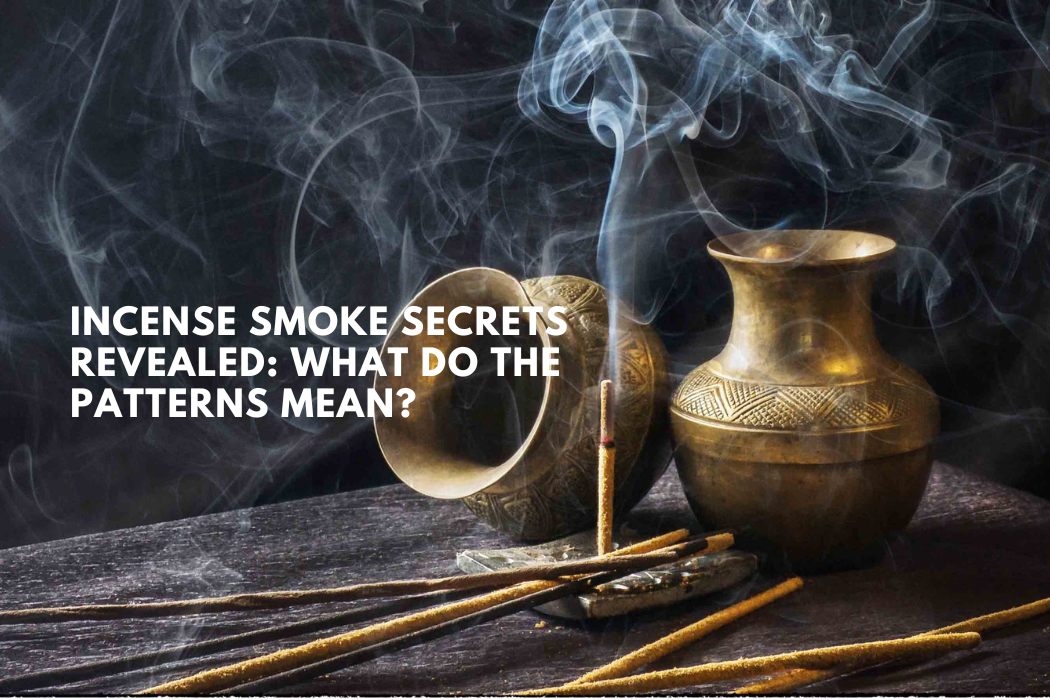**Detailed Caption:**

This professional photograph captures the serene and mystical moment of incense being lit. The central focus is a single stick of incense positioned delicately in a stylish incense holder, from which ethereal swirls of smoke ascend and drift gracefully across the image, creating an enchanting foreground effect. Nestled behind the incense, two intricately designed golden vases add a touch of elegance; one stands upright, while the other lies tilted, allowing a glimpse into its opening. Both vases feature a narrow neck that flares into a broad, rounded base. Scattered in the foreground are several more sticks of incense, lying at a casual angle on a dark, polished wooden table. Enhancing the dramatic atmosphere, the background is a deep, pure black. Overlaying the entire image, a thought-provoking headline in white text reads: "Incense Smoke Secrets Revealed: What Do the Patterns Mean?" The meticulous composition and the evocative elements suggest this photograph could seamlessly belong in a high-quality magazine article or an insightful blog post.